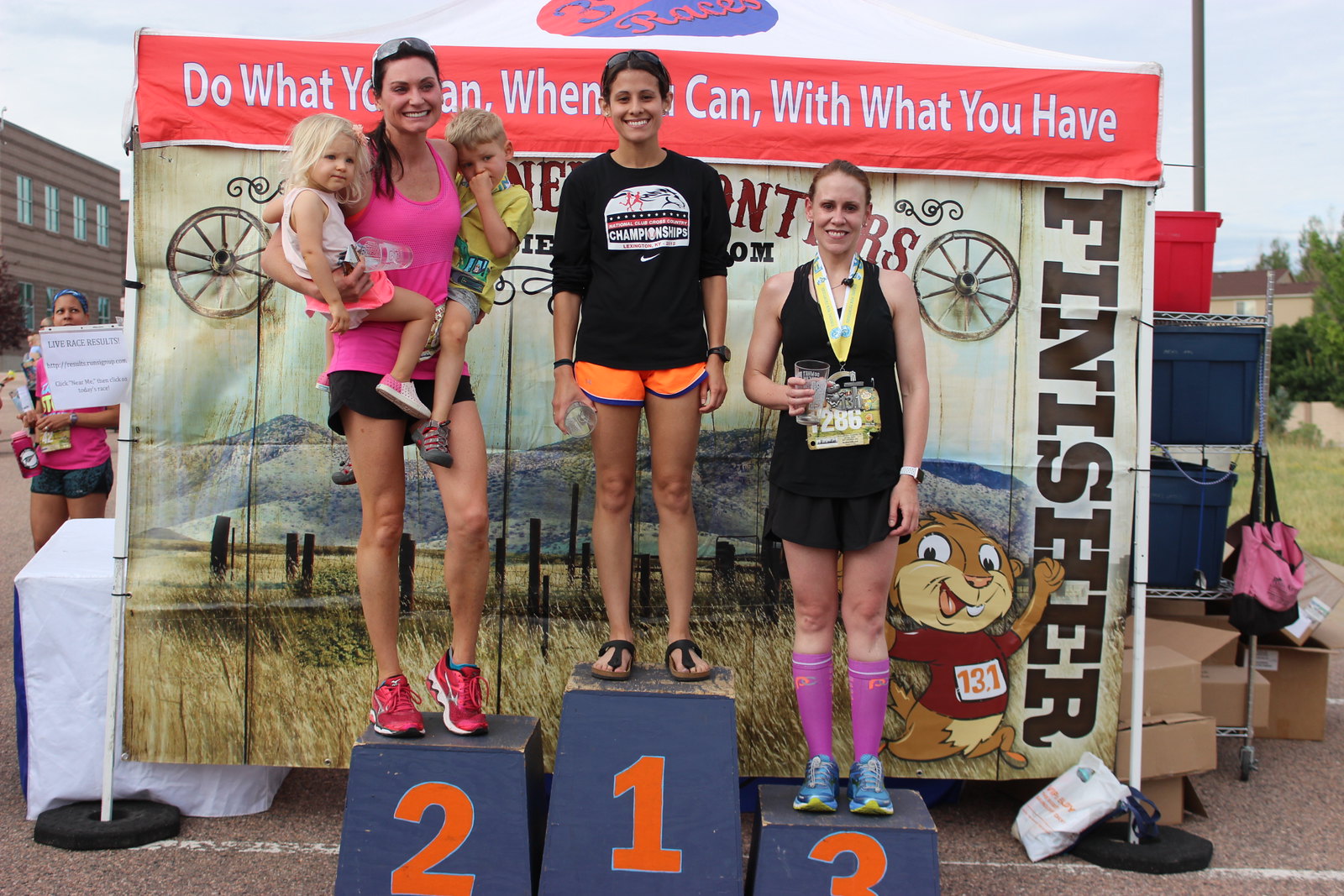In this vibrant outdoor photograph, three women stand proudly on a blue-painted podium, celebrating their achievements in a competition held on a sunny day. They are positioned in front of a backdrop displaying a scenic field and mountain landscape, adorned with a playful chipmunk illustration wearing a shirt numbered 131 and a large red banner proclaiming, "Do what you can, when you can, with what you have," partially obscured by their heads. 

The first-place winner, centered, captures attention with her broad smile, dressed in a black t-shirt adorned with a white design, complemented by orange shorts with blue trim and sandals. She holds an object in her right hand. 

To her right, on the second-place block, stands a fair-skinned brunette with dark hair and sunglasses perched on her head. She is dressed in a pink tank top, black shorts, and red shoes, while she balances a little blonde boy and girl in her arms—a boy in a green shirt and gray shorts, and a girl in a white top with a pink skirt. 

The third-place finisher, on the left, sports a black sleeveless shirt and black shorts, her race number 286 pinned to her front. She wears purple socks with tangerine details and blue tennis shoes, her right hand holding a cup and a lanyard hanging around her neck.

Behind them, a sign reading "finisher" and a table with a woman in a pink shirt, narrow glimpses of nearby buildings, and scattered crates are visible, framing this celebratory moment of achievement and camaraderie.